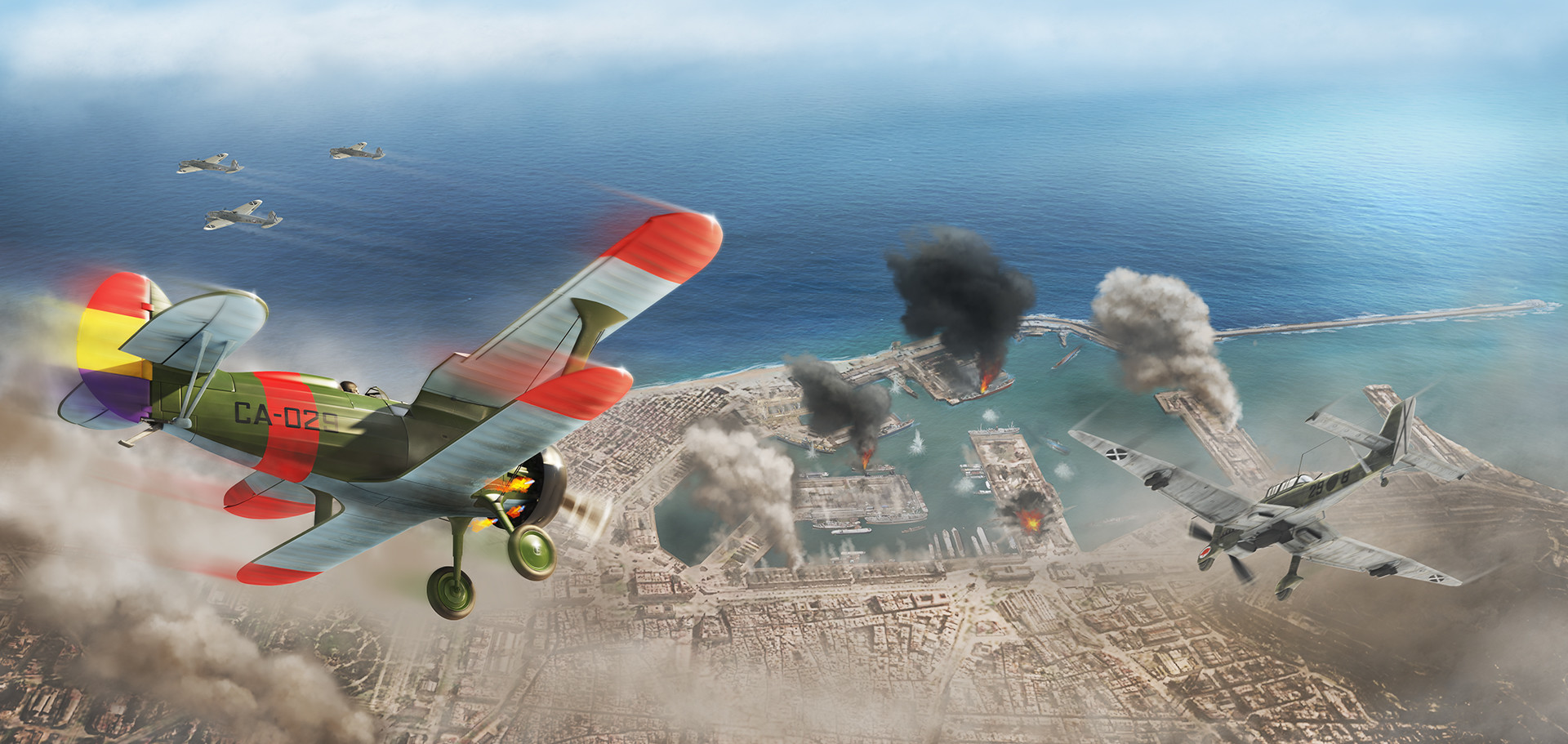A vibrant digital painting depicts a dramatic aerial dogfight scene against a backdrop of a blue sky and distant ocean. On the left, a distinctive biplane with a green body, blue wings tipped in red, and a tail adorned with red, yellow, and purple stripes, dives down with its propeller spinning. The plane is marked with "CA-025" in black text on the rear fuselage. To the right and slightly lower, a smaller, all-gray monoplane with a single wing and a propeller also flies amidst the fray. Both planes are surrounded by spiraling black, gray, and white smoke, indicative of the ongoing battle. Below the airborne chaos, an island city sits in grayscale tones, its roofs and ground interspersed with towering columns of light and dark gray smoke due to fires marked by bright red and yellow blazes. In the far distance over the blue expanse of the ocean, three additional gray planes with white, smoke-trailing wings can be seen flying in formation towards the upper left corner of the sky. Tiny ships dot the surrounding waters, barely visible from the height of the action-filled scene.